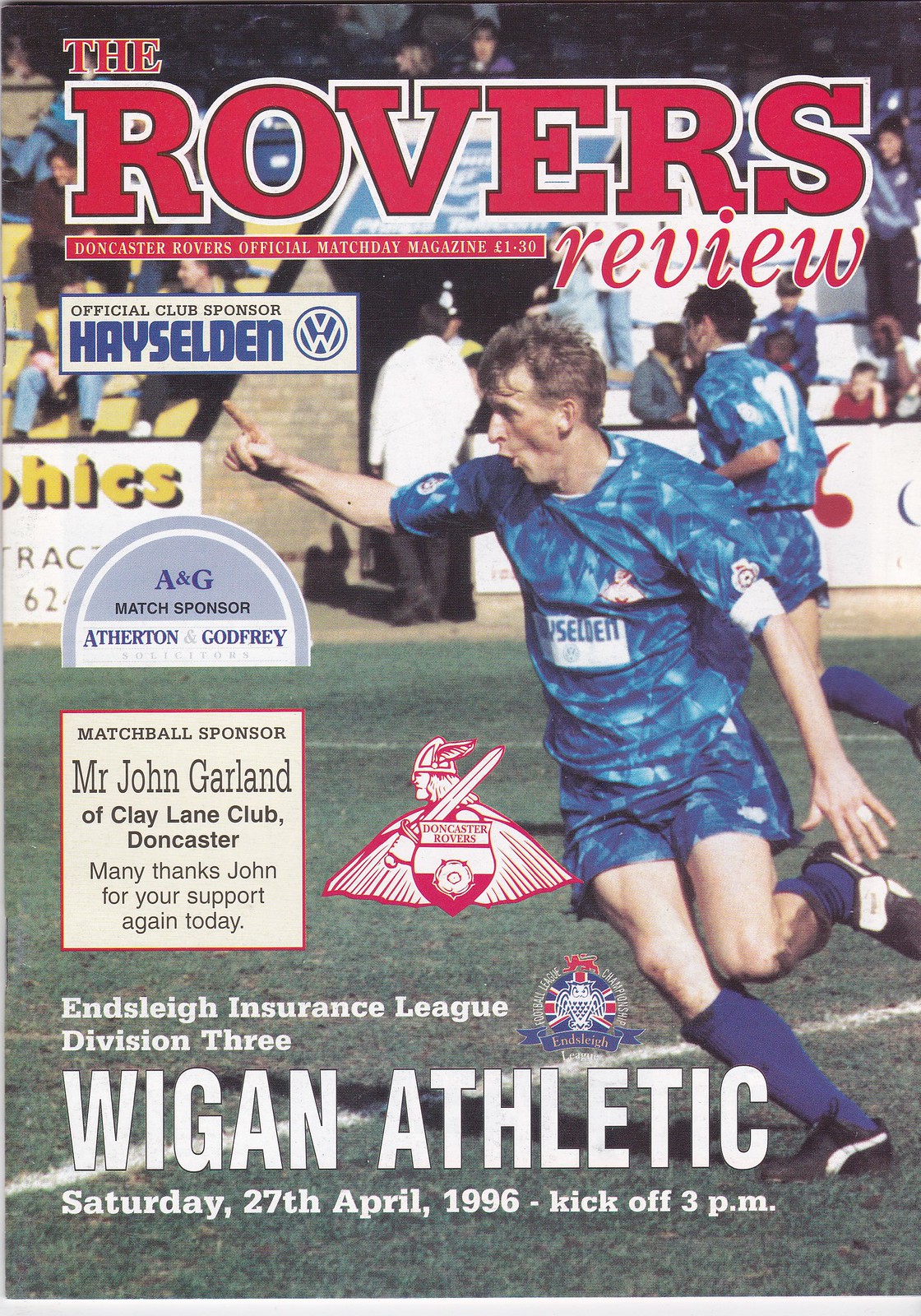The vertically aligned rectangular image is the cover of a magazine titled "The Rovers Review." The title "The Rovers" is emblazoned across the top in large, red all-caps letters with a white outline, with "The" appearing just above the "R" in smaller print. Below this, in smaller print, it reads "Doncaster Rovers Official Match Day Magazine 1-30," although the text is quite small. The word "Review," in lowercase red letters, is positioned under the "ERS" in "Rovers."

On the left side of the cover, several sponsors are noted. The "Official Club Sponsor Hey Selden" appears alongside the Volkswagen logo. Below this is "A&G Match Sponsor Atherton Godfrey," and further down in a white square outlined in red, it states "Match Ball Sponsor Mr. John Garland of Clay Lane Club Doncaster. Many thanks, John, for your support again today."

Toward the bottom left, it says "Ainslie Insurance League Division 3" in regular print, while "Wigan Athletic" is highlighted in all-caps large white letters. Below this, it specifies, "Saturday, 27 April 1996, kickoff 3 p.m."

Dominating the right side and center of the magazine cover is a photo of a soccer player running, adorned in blue and white shorts and jersey, blue socks, and black cleats. He is the focal point, with another player in the background moving in the opposite direction. The main player has his right arm outstretched, pointing ahead with his forefinger. In addition to the main image, there is a smaller graphic of a Trojan or Spartan warrior, equipped with a metal helmet adorned with wing-like decorations, a cape, a sword, and a shield. The scene is set against what appears to be a sunny day with a visible audience in the stands, adding to the lively atmosphere of the match.